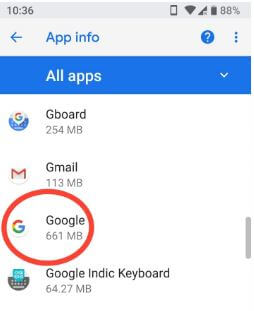This image is a low-quality screenshot from an older Android phone, showcasing the 'App Info' menu within the basic settings. At the top, a blue banner with the label 'All apps' is visible, indicating that the user can scroll down to view and select various downloaded apps to examine their information. The screenshot highlights several apps, each accompanied by their respective icons and the amount of storage they occupy. Among them, Gboard uses 254 megabytes, Gmail consumes 113 megabytes, Google takes up 661 megabytes, and Google Indic Keyboard uses 64.27 megabytes. A circular annotation is drawn around the Google app, suggesting that this screenshot may be part of a tutorial, likely instructing the user on how to access and manage the app info for Google. The time displayed is 10:36 (either AM or PM), the battery level is at 88%, and various status icons are present in the top right corner, offering further context on the phone's status.